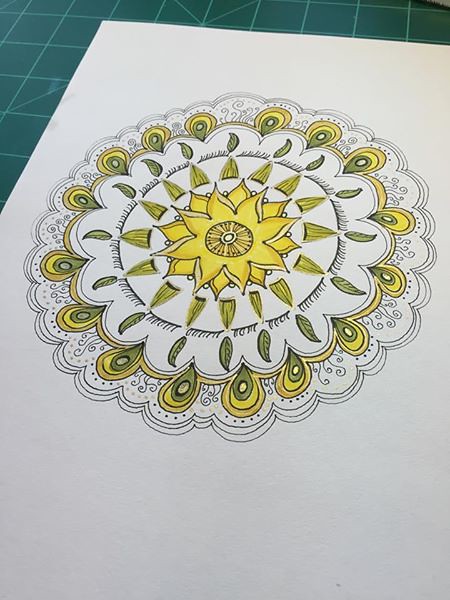The image captures a detailed drawing on white, unlined paper, showcasing an intricately designed geometric pattern. At the center, there is an eight-petaled sun or flower motif. Between these petals, additional overlapping petals emerge, creating a layered floral effect. Extending outward from this central motif are pointed leaves interspersed with lines and further leaves, forming concentric rings. The outermost layer features designs reminiscent of peacock feathers. The artwork is meticulously colored in shades of yellow and varying tones of green. The backdrop of the image includes a green grid typically used for artistic purposes, setting a structured frame for the drawing.